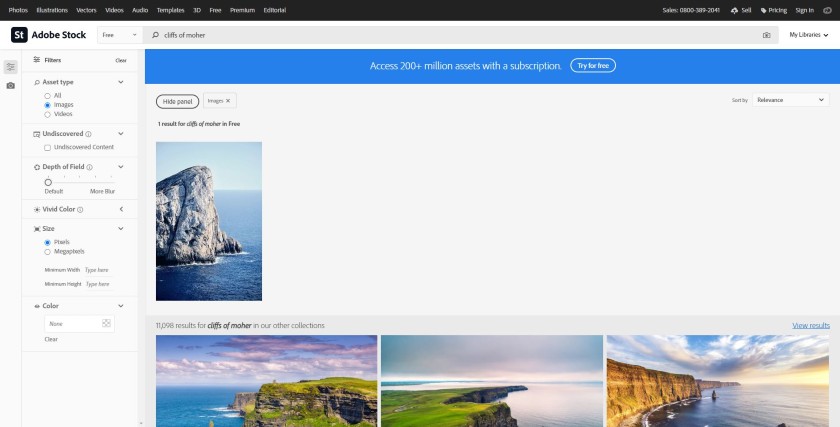This screenshot captures the interface of Adobe Stock's application. At the very top, there are various navigational links prominently listed in the top left corner, including "Photos," "Videos," "Audio," "Template," "Free," "Premium," and "Editorial." Centered at the top is a large search bar for easy browsing.

Just below the search bar, a blue banner spans the width of the page, featuring the text: "Access 200+ million assets with a subscription. Try for free."

In the center and bottom right of the image, four high-definition photographs are displayed, each showcasing picturesque edges of different islands set against open water, resembling oceanic scenes. These images are captured with a wide-angle lens, beautifully portraying the skies and horizon.

On the left side of the interface are various selectable options, suggesting functionalities related to photo editing or asset browsing. The page maintains a clean, all-white background characteristic of Adobe's design aesthetic.